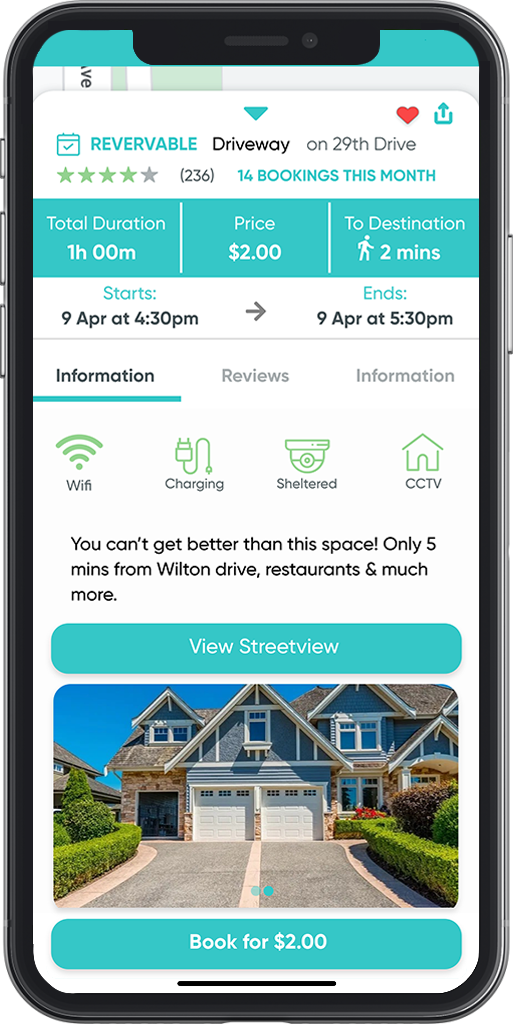A detailed description of the phone screen and its elements:

The phone in the image has a black outline with a silver button on the front. On the left-hand side are three buttons, and on the right-hand side is one silver button. The screen displays a detailed interface.

At the top of the screen, there is a teal-colored line running across, resembling a tail. Below this line, the screen appears to display a map, but it is largely obscured by a white pop-up window. On the map, the word "Avenue" can be deciphered from partially visible letters "VE" on a black background.

Within the pop-up, which occupies the majority of the screen, the following details are visible:
- At the very top in teal, it says "REVERVABLE."
- Below that, in black text, it reads "driveway."
- Further down, it says "on 29th Drive" in black letters, accompanied by a red heart above the word "Drive."

Beneath this text, there are star ratings indicating four green stars and one gray star, suggesting a 4 out of 5-star rating from 236 reviews.

In teal text, there is a mention of "14 book month." Following this, there is a teal rectangle banner dividing the screen into three sections:
1. On the left, the total duration is displayed as "1H 00M" (one hour).
2. In the middle section, the price is shown as "$2.00."
3. On the right, the estimated time to the destination is indicated by a white stick figure walking with "2 MINS" (two minutes) next to it.

Below this section, on a white background, the timing details for an event are listed. It states:
- The event starts on "9 APR at 4:30 PM" (in black text).
- The event ends on "9 APR at 5:30 PM."

A gray line separates this information from further details labeled "information" and "reviews information." Additional amenities listed include:
- Wi-Fi
- Charging
- Shelter
- CCTV

The description concludes with a promotional statement: "You can't get better than this space, only five minutes from Wilton Drive, restaurants, and more."